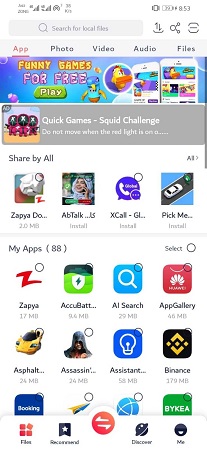The image features a predominantly white background, which serves as a clean canvas for the variety of elements it displays. Centered at the top is a prominent white box adorned with letters, presumably a title or label, followed by a search box equipped with up and down arrows for navigation. Adjacent to these elements is a distinct, small circle with two protruding extensions resembling arms, and a square icon containing a minus sign.

Below this section, there are tabs labeled "app," "photo," "video," "audio," and "files," each probably representing different categories or functionalities. An eye-catching, cartoonish background advertises "funny games for free," accompanied by a green play button featuring miniature character illustrations. These characters are vibrantly colored in blue, orange, and purple hues.

Further down, a purple box draws attention with the text "Quick Game Squid Challenge: Do not move when the red light is on," underscored by small purple characters positioned on the left side. This gaming prompt adds a dynamic and engaging element to the image.

In another white box, the options "share by all," "Zapya," "Do," "AppTalk," "Xcal," "PickMe," and "Line" are listed. Below this, "MyApps88" includes links to various apps like "Zapya," "Acubat," "AI Search," "AppGallery," "Asphalt," "Assassin," "Assistant," "Finance," and "Booking." Noteworthy icons include one resembling a paper plane, and another depicting a blue globe. The green-labeled "Bykea" is also mentioned, delineating a specific app or service.

Towards the bottom, a black flag with a white star, a red circle with white marks, options labeled "discover," and "me" appear, featuring additional navigation or profile options.